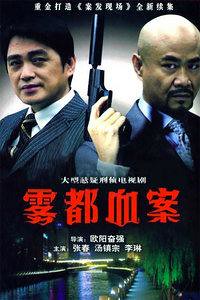The image is a Chinese movie poster featuring two men of Asian descent standing back-to-back. The man on the left has dark black hair, is clean-shaven, and is wearing a gray pinstriped suit with a white shirt and black tie. He has a slight smile on his face. The man on the right is bald with a black French beard and mustache, wearing a blue suit, blue shirt, and blue tie. He is holding a large black gun with a silencer in his right hand, which is prominently displayed between the two men. The scene appears to depict only their upper bodies. 

Above the men, there are Chinese characters, and below them are multiple lines of Chinese text. The largest text is in red, likely indicating the title of the movie. Beneath that, there are additional lines of Chinese text in white, in progressively smaller fonts.

At the bottom of the poster, there is an image of an outdoor nighttime scene that includes a road, some trees, tall reedy grass, water, and buildings in the background. The overall composition splits the image, emphasizing both the men and the Chinese text.